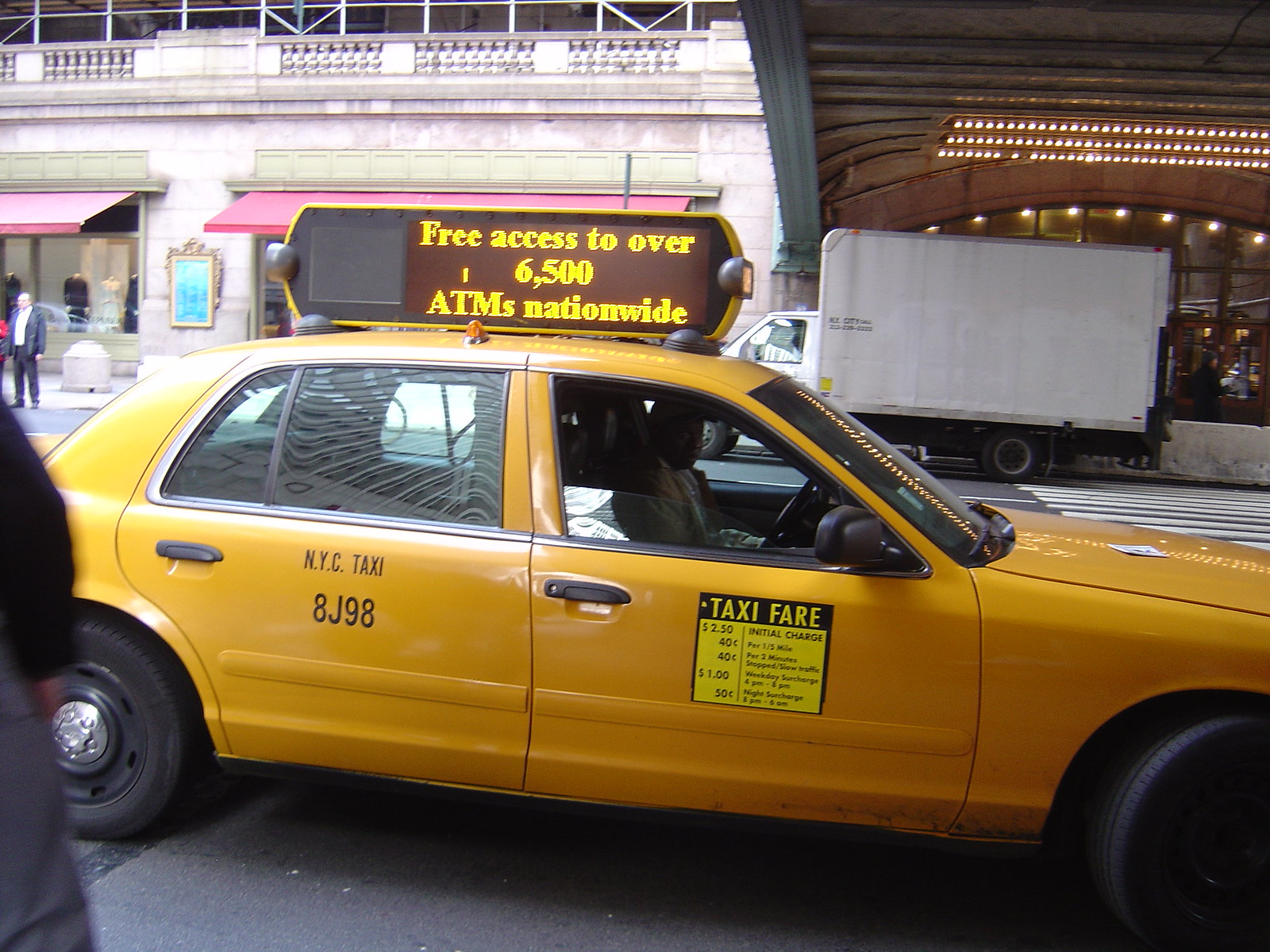This photograph captures a bright yellow New York City taxi cab, numbered 8J98, at a stop along a dark gray pavement street. The cab, a four-door sedan, is positioned facing left to right, though the front and rear ends are slightly cropped out of the frame. The driver, visible but indistinct in the dim lighting, faces the camera, and the front passenger window is rolled down while the rear window remains up. On the roof of the taxi, an advertisement reads, "Free access to over 6,500 ATMs nationwide." The fare details are prominently displayed on the front passenger door, listing an initial charge of $2.50, 40 cents per half mile or two minutes, a $1 weekday surcharge (4 p.m. to 8 p.m.), and a 50 cent night surcharge (8 p.m. to 8 a.m.). The clean, shiny vehicle has a piece of paper casually discarded on its hood. In the background, a grand grey stone building with red awnings and a balcony stands to the left, while a sage green-trimmed bridge extends to the right. Further back, a white box truck travels in the opposite direction of the taxi, beneath rows of lights. The composition suggests an urban scene bustling with activity.